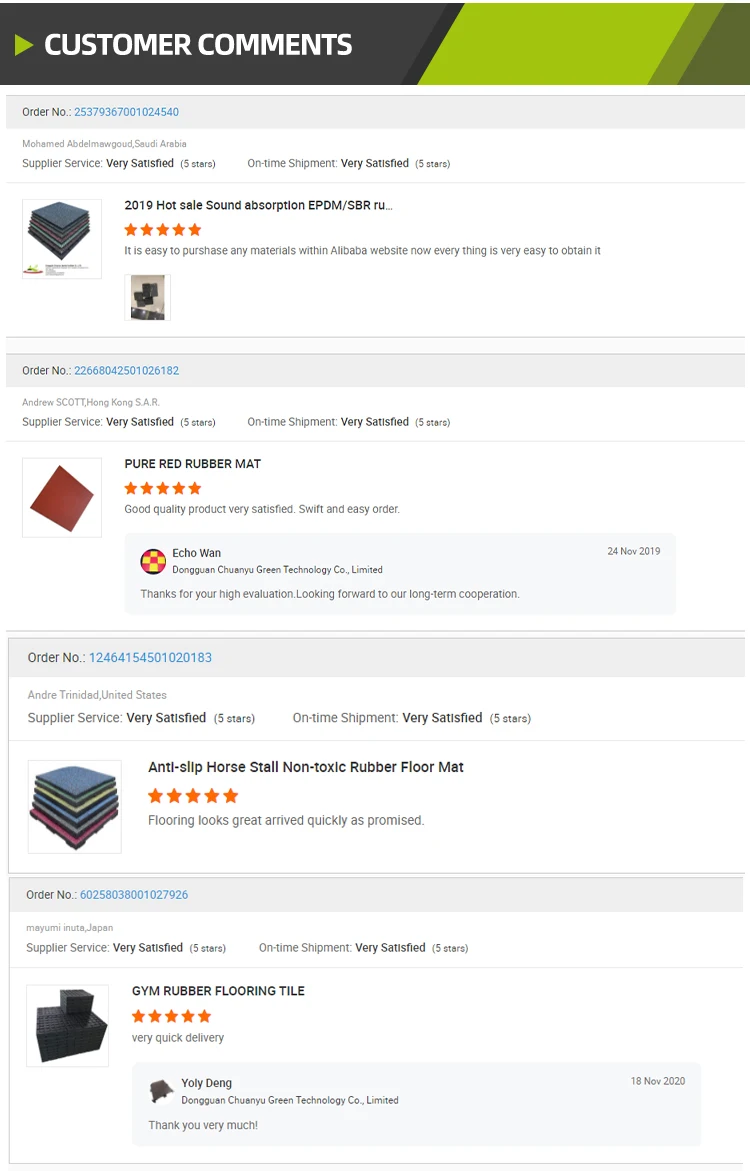The image captures a mobile phone screen displaying customer comments on their recent purchases from Alibaba. At the top of the screen, an order number is highlighted in blue. Beneath it, the customer details their purchase of a "2019 Hot Sale Sound Absorption EPDM/SBR." The comment mentions how easy it is to purchase materials through the Alibaba website, alongside a visual of sound absorption padding composed of interlocking squares.

As you scroll down, the next order number appears along with the customer name, Andrew Scott from Hong Kong SAR. This comment praises the supplier's service and satisfaction with the purchase of a "Pure Red Rubber Mat," describing the product as high quality and the order process as swift and easy.

Further down, another order includes an "Anti-Slip Horse Stall Non-Toxic Rubber Floor Mat." The customer notes that the flooring looks great and arrived quickly as promised. Finally, the comment section highlights the purchase of "Gym Rubber Flooring Tile," for which the customer expresses their satisfaction with the very quick delivery, awarding it five stars and adding a "Thank you very much" at the bottom.